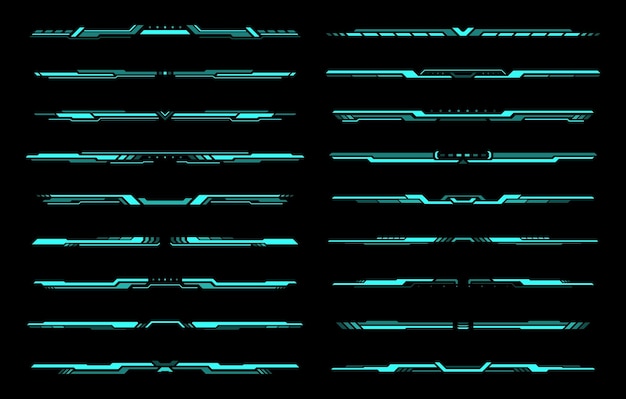The image is a computer-generated rendering featuring a plain black background. Displayed prominently are two columns of teal-blue lines, each column containing nine lines. These lines exhibit a low-level neon glow, highlighting the teal-blue color. The lines are not uniform; each one is distinct with varying geometric shapes, some resembling car grill work or pinstriping, and others akin to pilot wings on a uniform. The structures are composed of long, thin rectangles, dashes, or dots, creating a complex interplay of shapes. There are spaces between these elements, allowing the black background to show through. Notably, most lines have a protrusion or some form of discontinuity in the middle, except for a few straight lines such as the second in the first column and the eighth in the second column. Overall, there is no labeling or identification on the slide, leaving the visual elements to speak for themselves.